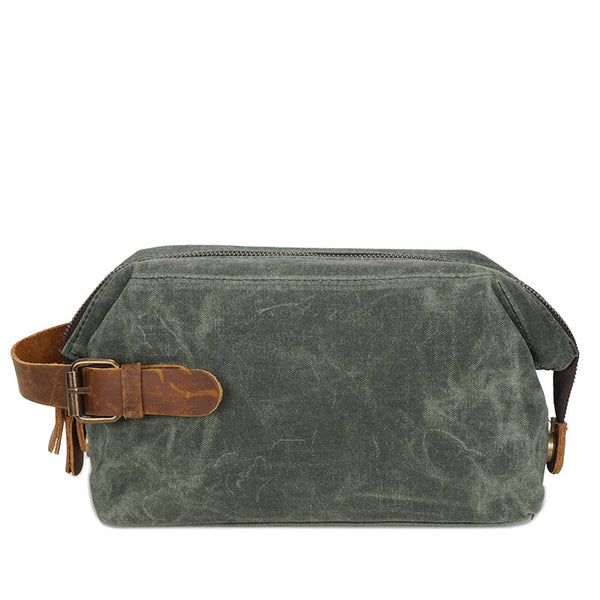This is a color photograph of a small, rectangular satchel or bag, likely intended for travel or toiletry use, rendered in worn, suede-like material. The bag features a distinct, desaturated gray-green hue with subtle yellow undertones, showing visible signs of distress along its edges, characteristic of suede fabric. At the top of the bag, a zipper spans from the top left to the top right, with the ends of the zipper causing the bag to slump slightly at the edges, possibly due to wear or design intent. A brown leather strap with a belt buckle accent is affixed to the left side of the bag and loops around to the back, but its exact reattachment point is not visible. There may be a similarly colored leather tag or fringe detail adjacent to the strap. The photograph is set against a plain white background, where the bag's edges exhibit some fuzzy, less refined Photoshop work compared to the crisper top and other edges. The photo is devoid of any writing, people, animals, or structures, keeping the focus solely on the bag itself.